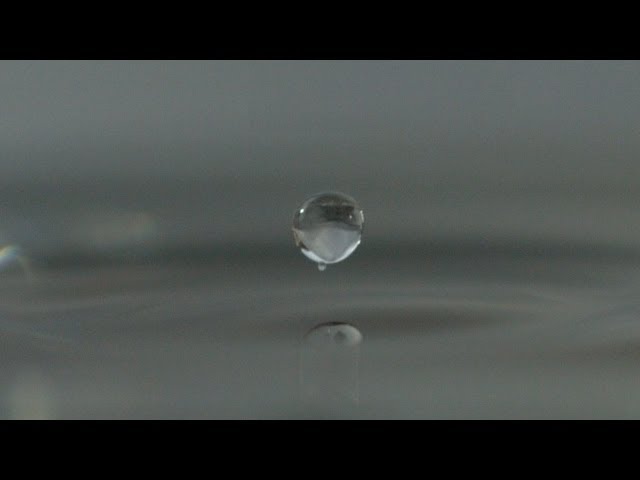This still image, formatted in a 16:9 aspect ratio with black bars at the top and bottom, depicts a clear and reflective water droplet poised in mid-air, just moments before impacting the grayish body of water below. Central to the composition, the translucent droplet is almost spherical and exhibits a subtle reflection within its structure, hinting at its clarity and purity. Beneath the primary droplet, a smaller connected droplet can be observed, emphasizing the impending collision with the water surface, which already shows the residual circular ripples from previous droplets. The overall gray tone of the image, coupled with the white highlights on the droplet, grants it a shimmering, almost diamond-like quality, beautifully encapsulating the delicate moment just before the water disturbance.